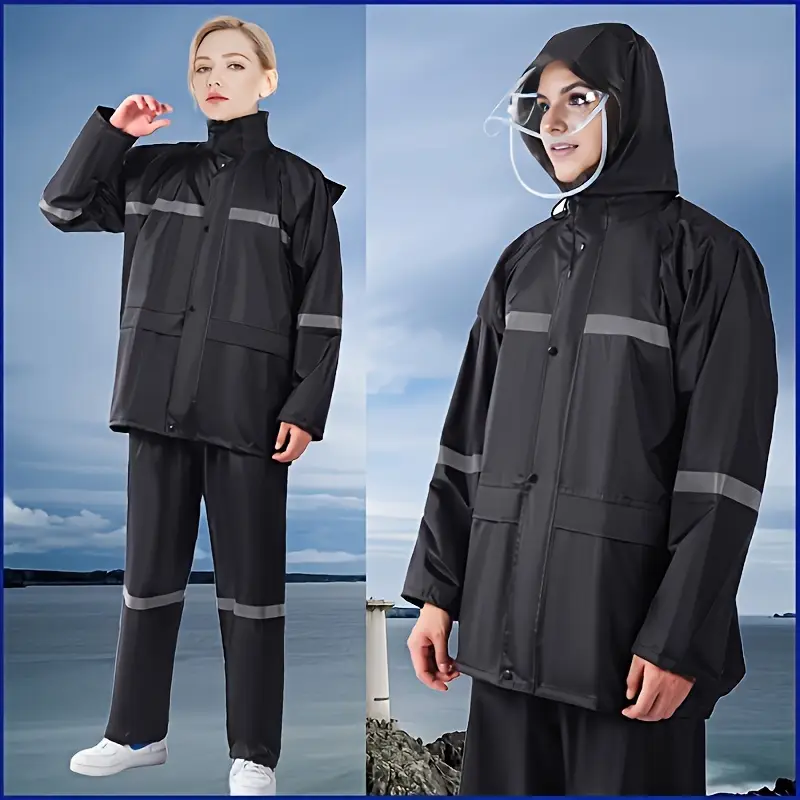The image is a highly stylized fashion magazine shoot featuring two variations of a female model, depicted with a vertical separation between the images. Both females are dressed in dark black or grey waterproof rain gear, consisting of a two-piece jacket and trousers ensemble. Reflective silver or grey stripes are artfully placed around the knee, elbow, and chest areas, adding visual interest and highlighting the garment's functionality. The model on the left, who has blonde hair tied back and very pale skin, is posing with her right hand up towards her face and her left hand at her waist, looking directly into the camera. Her jacket, featuring storm flaps, large pockets, buttons, and a zip, pairs seamlessly with her plain white trainers. She is photoshopped against a surreal background of a dark grey-blue water surface and a sky filled with horizontal cloud layers, creating an impression of her standing on water.

On the right, the same model wears an identical outfit but with the hood raised. Her hands are down by her sides, and she gazes off into the distance to the left of the frame. The hood includes a light plastic visor trimmed in white, providing additional protection from the elements. This image is also photoshopped, showing her against a slightly different background that suggests an oceanic theme complete with rocks, water, and what could be a lighthouse in the distance. Both halves of the composition use artificial, dreamlike backdrops to enhance the chic, modern aesthetic of the waterproof fashion line being showcased.